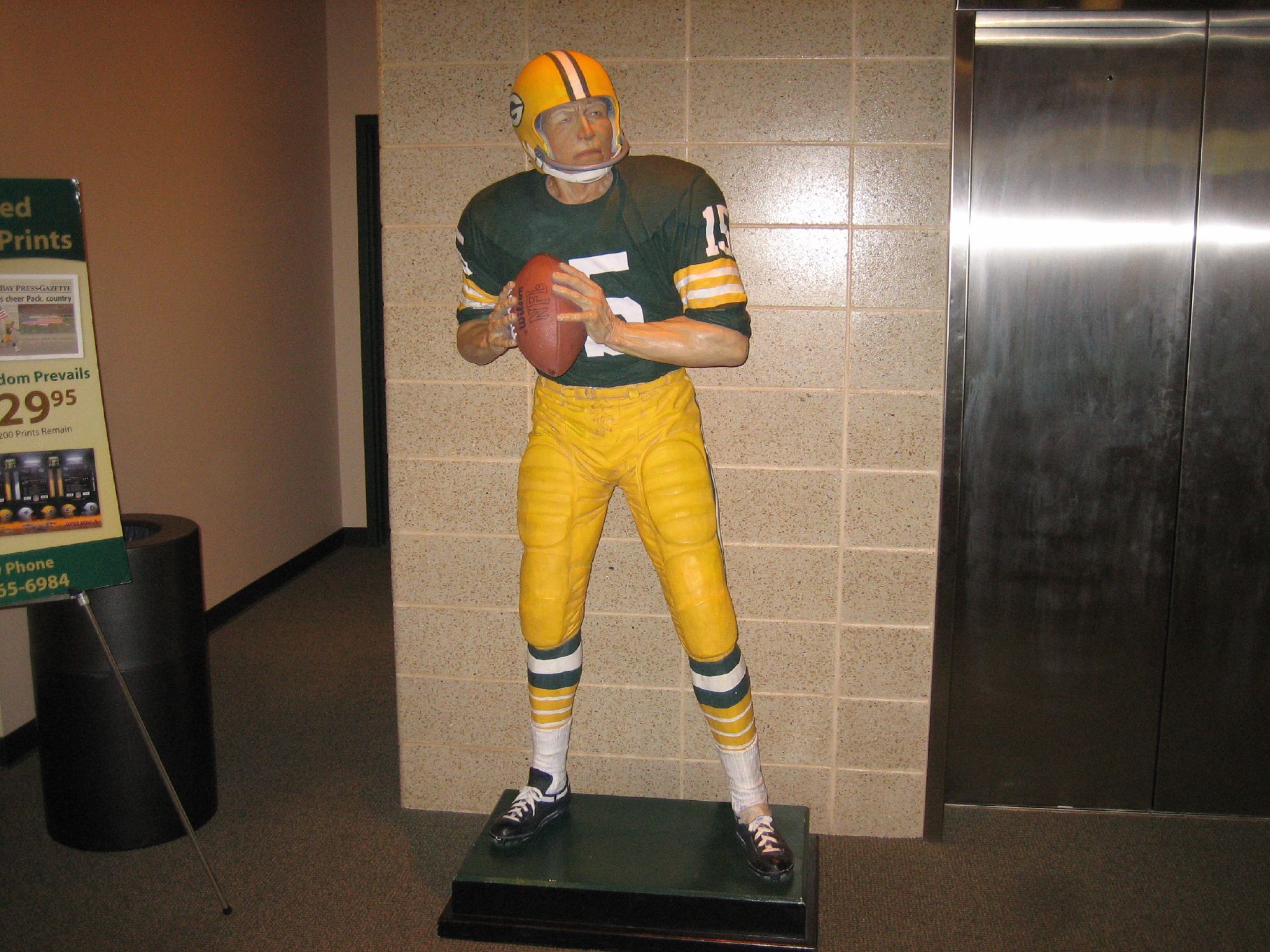This detailed photograph captures a life-size statue of a Green Bay Packers football player positioned inside what appears to be a convention center or lobby. The statue features an old-fashioned uniform, characterized by a yellow helmet with the Green Bay Packers' G logo and a single-bar face mask, complemented by a white and green stripe down the middle. The player is wearing a green jersey with the number 15, yellow pants, and green, white, and yellow striped socks paired with black cleats. He holds a red football in both hands, poised as if looking slightly to the right, ready to throw it downfield. The statue stands on a rectangular dark green and black platform. Surrounding the statue, there is a cream-colored wall made of rectangular tiles in the background. To the left of the statue, a cylindrical-shaped trash can and a board are visible, while to the right, silver elevator doors indicate the presence of a gate that looks like an elevator entrance. The entire setup suggests a blend of nostalgia and tribute, encapsulated within this specific hallway area.